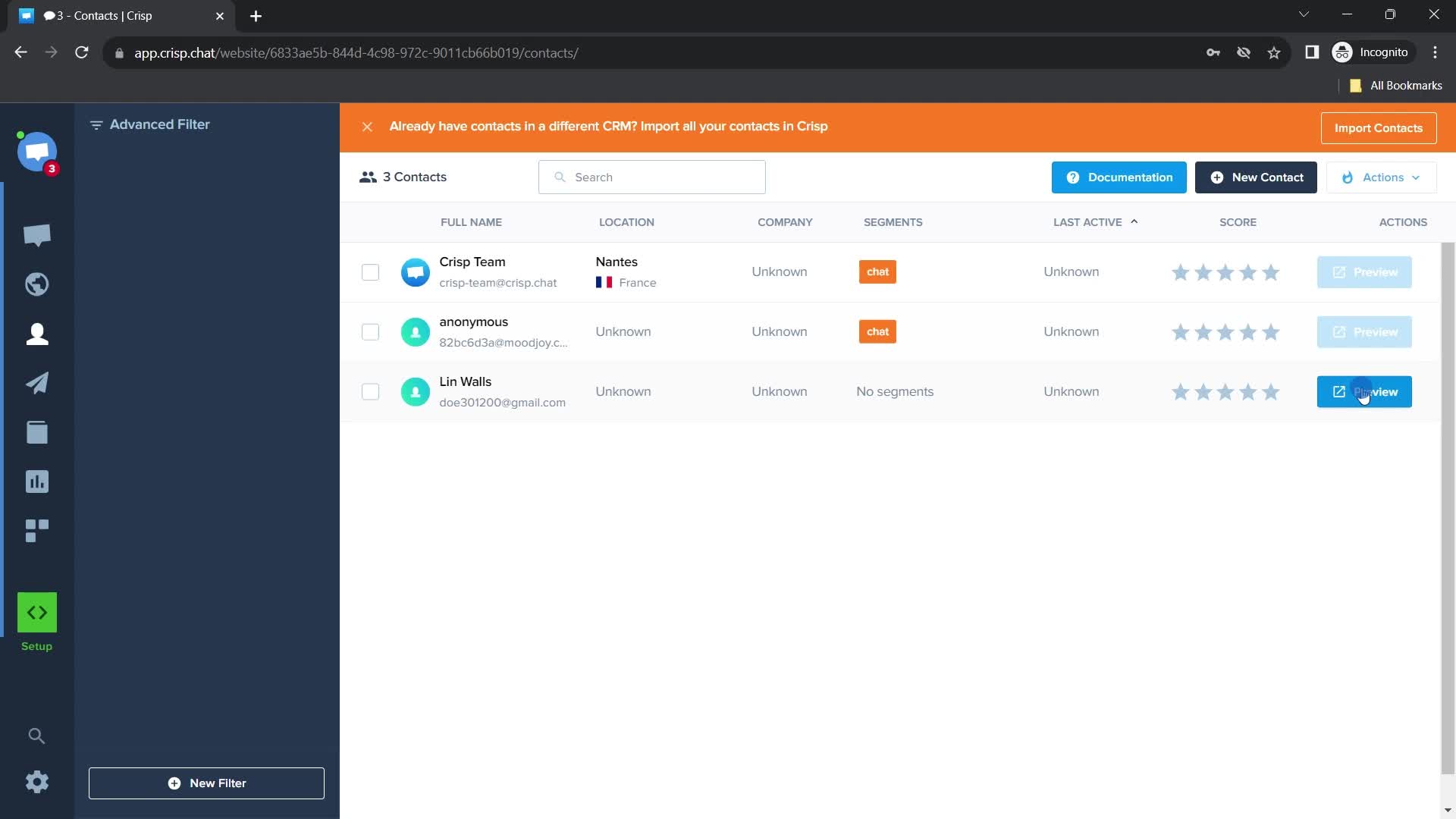In the image, we see a detailed screenshot of a web application. At the top, there is a black header which features white text in the upper left corner that reads "Three Contacts - Crisp." Below this header, there is a black address bar displaying the URL "app.crisp.chat/websites."

Continuing down the left side of the screen, there is a vertical toolbar. The toolbar is topped by a blue circle with a white message icon inside it, a small number "3" in white, and a red circle at the bottom of the blue circle. Below this icon, there are other icons representing a globe, a text message, and a document. At the bottom of this toolbar, there is a green box with the word "Setup" written below it.

To the right, occupying the main portion of the screen against a white background, there is a box listing three contacts. The contacts are listed one after another: "Crisp Team" at the top, followed by "Anonymous," and then "Lynn Walls." For each contact, there are columns providing detailed information including "Full Name," "Location," "Company," "Segments," "Last Active," "Score," and "Actions."